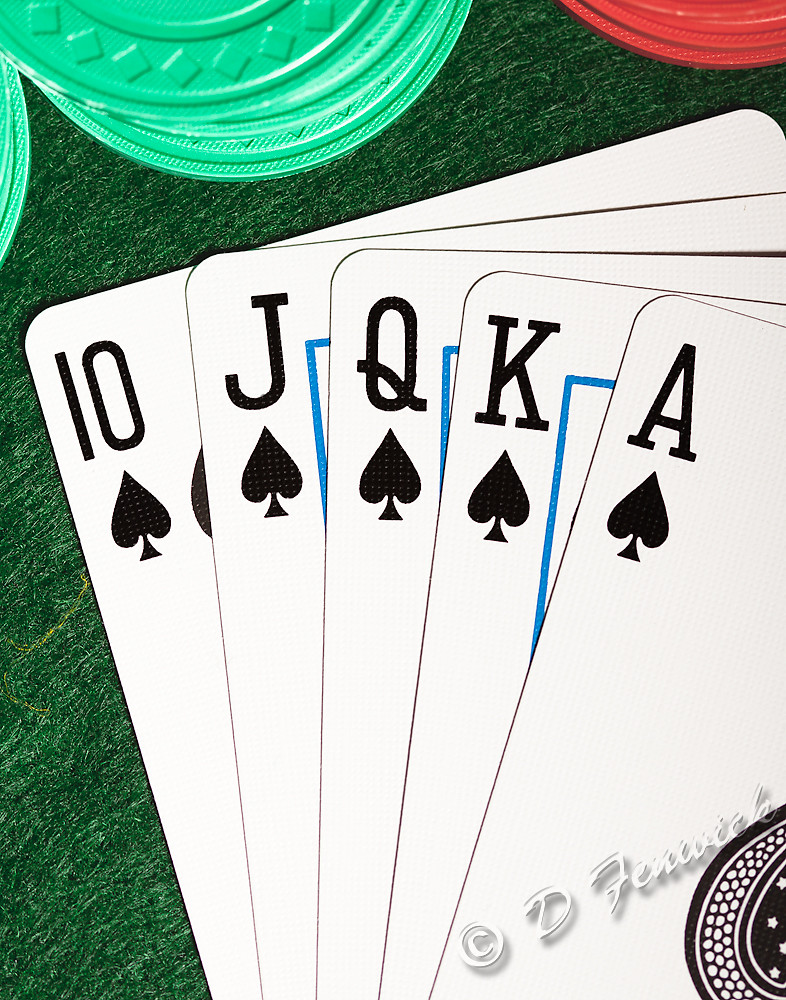This detailed caption describes an image featuring a poker scene:

In this meticulously detailed image, five playing cards are arranged in a fan-like manner, revealing a flush in spades from ten to eight. The cards are displayed across a green felt surface, often found on poker tables. The backdrop adds to the atmosphere with two stacks of medium green poker chips and one stack of red chips, hinting at an ongoing poker game. A white logo in the bottom corner states "Copyright D. Vexwick," suggesting that this may be a work by the artist, although it's ambiguous whether the image is a photograph or a digitally altered drawing. This visual composition effectively captures the essence of a high-stakes poker game, highlighting a strong hand with a spades flush.